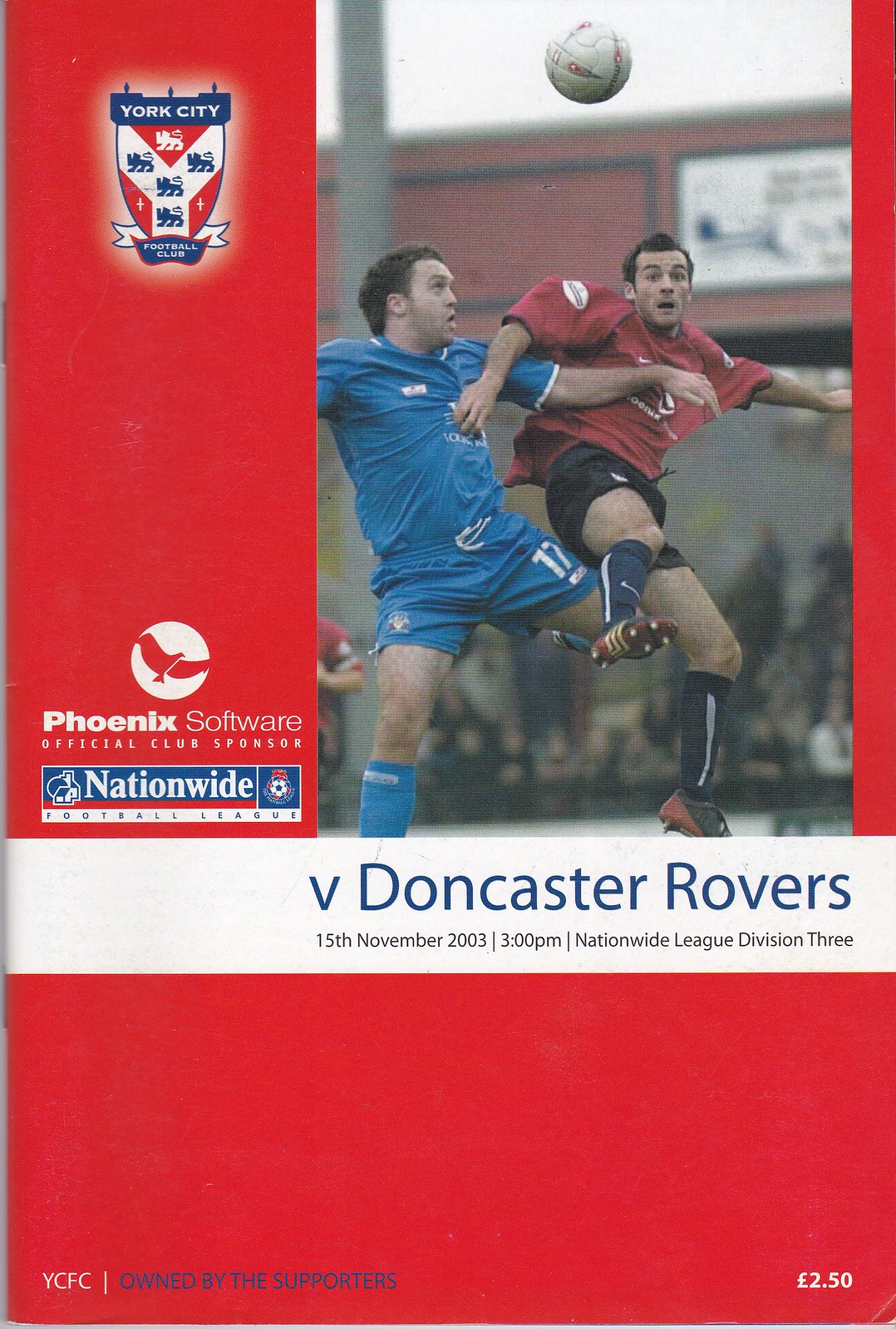This detailed caption synthesizes the key points from each contribution, highlighting common details:

The image is a cover of a program for a soccer match or football match in the UK between York City Football Club (YCFC) and Doncaster Rovers. The event took place on 15th November 2003 at 3 p.m., as part of the Nationwide League Division III. The top left corner of the cover features the York City Football Club seal, depicting a red and white shield. The background is predominantly bright red.

Central to the cover is a dynamic photograph of two players competing for the ball, which is suspended high in the air. The player on the left is clad in a blue shirt, shorts, and socks, looking upwards at the ball. His opponent on the right wears a red shirt with black shorts and socks and is looking straight ahead. Their legs appear intertwined, emphasizing the intensity of the struggle for possession.

Beneath the photograph, blue letters read "versus Doncaster Rovers.” Additional match details follow: "15th November, 2003, 3 p.m., Nationwide League Division III." The main sponsors, Phoenix Software and the Nationwide Football League, are also mentioned on the cover. At the bottom left, it states, "YCFC owned by the supporters," and on the bottom right, the program's cost is listed as £2.50.